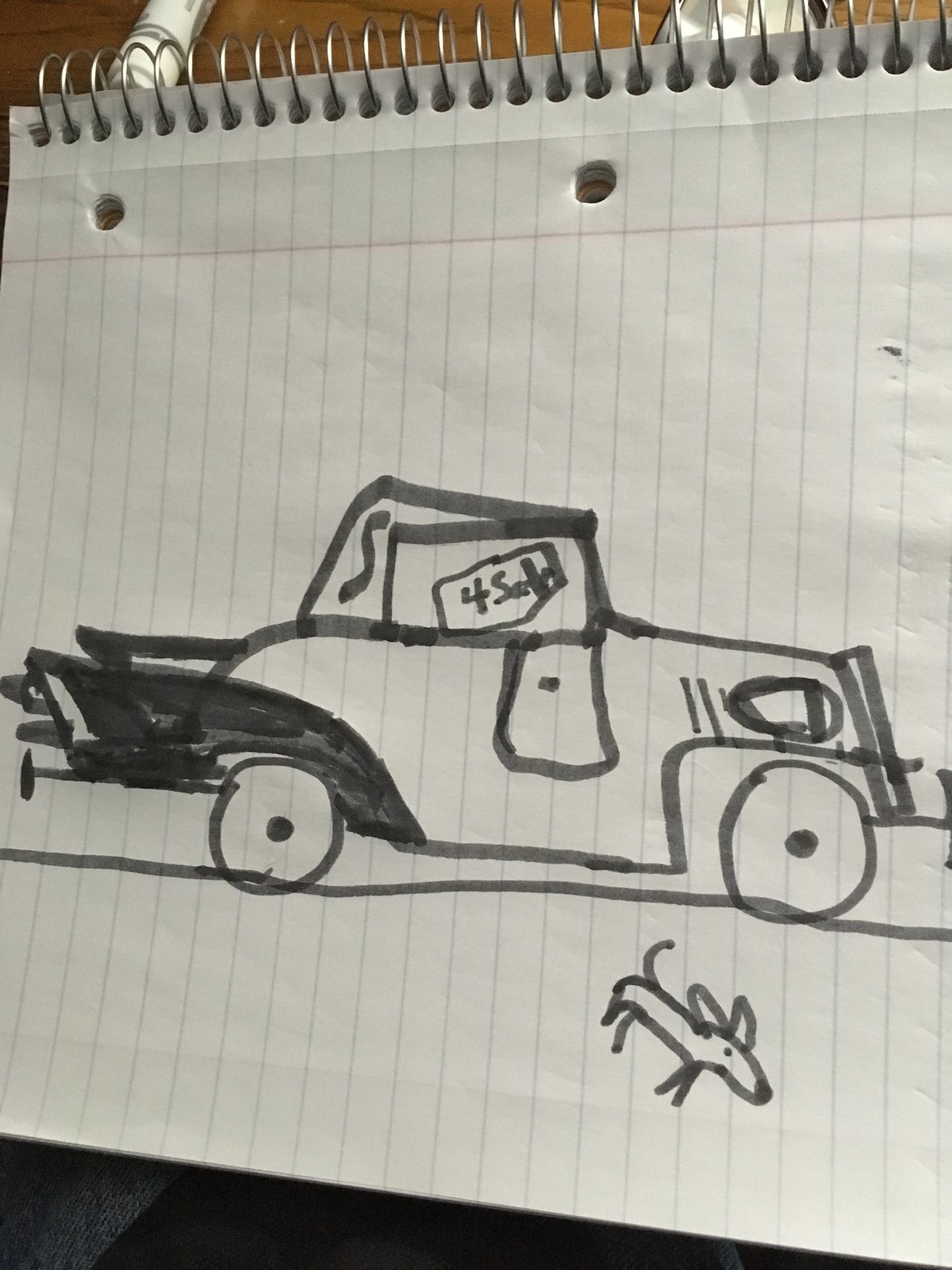This charming illustration presents a child’s artistic depiction of a vintage car. Rendered in marker on spiral-bound notebook paper, the drawing spans horizontally, effectively making use of the portrait orientation. The car portrayed is reminiscent of early 1920s or 1930s models, featuring a single door and adorned with both front and rear fins. Notably, there is a visible tailpipe and a single headlight on the front side. A distinctive "For Sale" sign is nestled in the window, although lacking any price information. A meticulously drawn grille and what appears to be a front crank add to the car’s antique charm. 

Complementing the scene, a simplistic black line across the page signifies the road on which the car rests. Along this road, a delightful stick-figure dog trots from right to left. The dog’s elongated body resembles a hot dog, complete with a curly tail, pointed ears, a single dot for an eye, and a noticeably long snout. This endearing image captures both the whimsical nature of children's artwork and a nostalgic nod to classic automotive design.